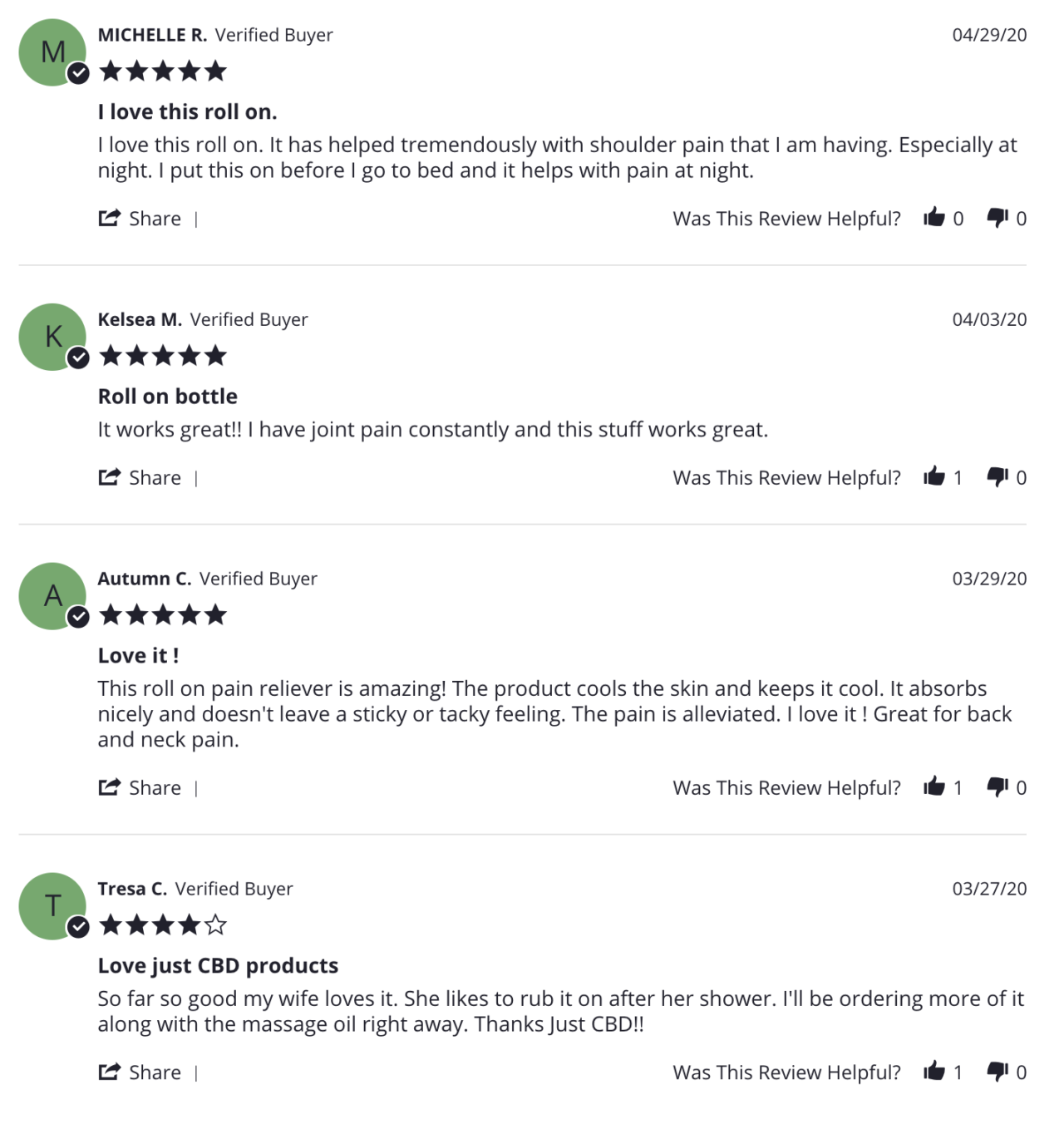In the image, there are four customer comments prominently displayed, each offering praise for a roll-on pain relief product. 

- The **top comment**, located at the top right corner, is from Michelle R., a Verified Buyer, who posted on April 29th, 2020. Michelle expresses her satisfaction, stating: "I love this roll-on. It has helped me tremendously with shoulder pain, especially at night. I apply this before bed, and it significantly reduces my nighttime pain."
 
- **Below Michelle's comment**, Kelsey M. gives a five-star review titled "Roll-On Bottle." Posted on April 3rd, 2020, Kelsey enthusiastically writes: "It works great!! I have constant joint pain, and this stuff is a game-changer."

- **The third comment** from the top is from Autumn C., also giving a five-star rating. Autumn posted on March 29th, 2020, and her review reads: "I love it! This roll-on pain reliever is amazing! It cools the skin, absorbs nicely without any sticky or tacky feeling, and effectively alleviates pain. It's great for back and neck pain."

- **The final comment at the bottom** is by Tersa C., who rated the product four out of five stars. Posted on March 27th, 2020, Tersa shares: "Love Just CBD products. So far, so good. My wife loves it and uses it after a shower. We'll be ordering more, along with the massage oil, right away. Thanks, Just CBD."

The bottom three comments all have a thumbs-up icon, indicating user approval, while the top comment from Michelle R. does not have this icon.